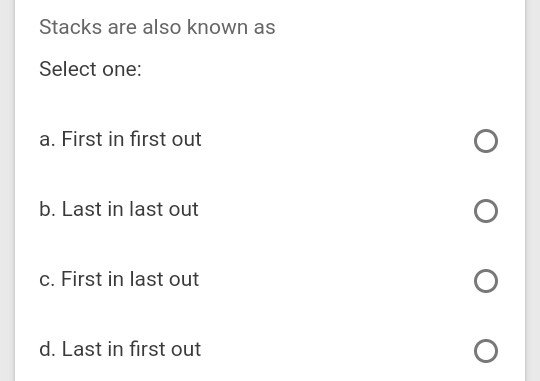In this image, we see a clean, white-background screenshot from a quiz application related to computer coding. The main area is bordered by two vertical gray lines on the left and right sides. Between these lines, there is a textual question that reads, "Stacks are also known as:", with "Stacks" capitalized.

Below the question, there are four answer options, each prefixed with a letter (A, B, C, D) followed by a period:
A. First In, First Out
B. Last In, Last Out
C. First In, Last Out
D. Last In, First Out

Each of these options has a corresponding empty circle to the right, indicating a clickable selection area for the user to choose their answer. Overall, the layout and design suggest that this is a user-friendly interface, likely part of a quiz or educational platform aimed at teaching coding concepts.